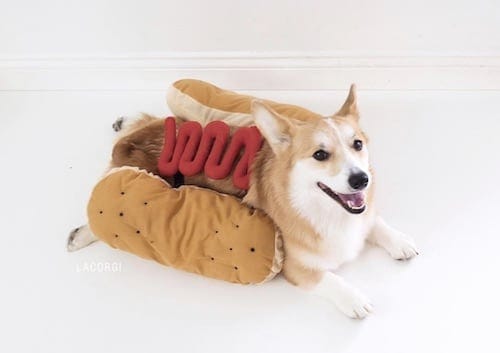A cheerful Welsh Corgi lies on a white floor, dressed in an adorable hot dog costume. The little dog's fur transitions from white at the face and neck to gold and finally a darker brown toward its back. The costume features bun-shaped pillows on either side of its body with a whimsical red squiggle representing ketchup running down its back. The Corgi's front legs are splayed out in front of it, and its back legs stretch out in the opposite direction. With alert, upright ears, sparkling black eyes, and an open mouth revealing his teeth, the dog looks directly at the camera, giving off a happy and playful demeanor. The background shows a white floor with the bottom edge of a wall and baseboard slightly jutting outward, suggesting the setting is likely someone's home.